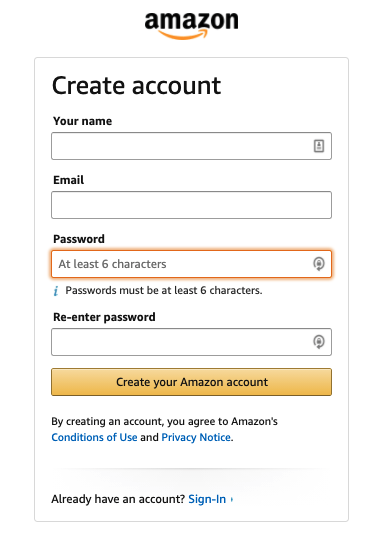In the image, there is a clean white background with the Amazon logo prominently displayed at the top, featuring the recognizable orange "swish" arrow. Below the logo lies a form enclosed within a white box, bordered by a light blue outline. This form is titled "Create Account" and is organized into several fields for user input.

The first field is labeled "Your name" with a text box provided for input. Adjacent to this text box is a small icon resembling an exclamation point, which likely serves as an error or alert indicator. The next section is for "Email," which also includes a text box for input.

Further down, the form includes a "Password" field, with the text box highlighted in yellow and red, indicating that extra attention is needed. A note within this field states "at least 6 characters," accompanied by a small circle and an indistinct symbol inside it. Additionally, there is a tiny "i" icon next to it, which provides a tooltip when hovered over, stating "passwords must be at least 6 characters."

Following the password field, there is another section labeled "Re-enter password" with a corresponding text box and similar circle-icon combination. 

At the bottom of the form, there is a prominent orange button labeled "Create your Amazon account." Beneath this button, fine print reads, "By creating an account, you agree to Amazon's Conditions of Use and Privacy Notice." Lastly, at the bottom of the form, a link is provided for users who already have an account, reading "Already have an account? Sign in."